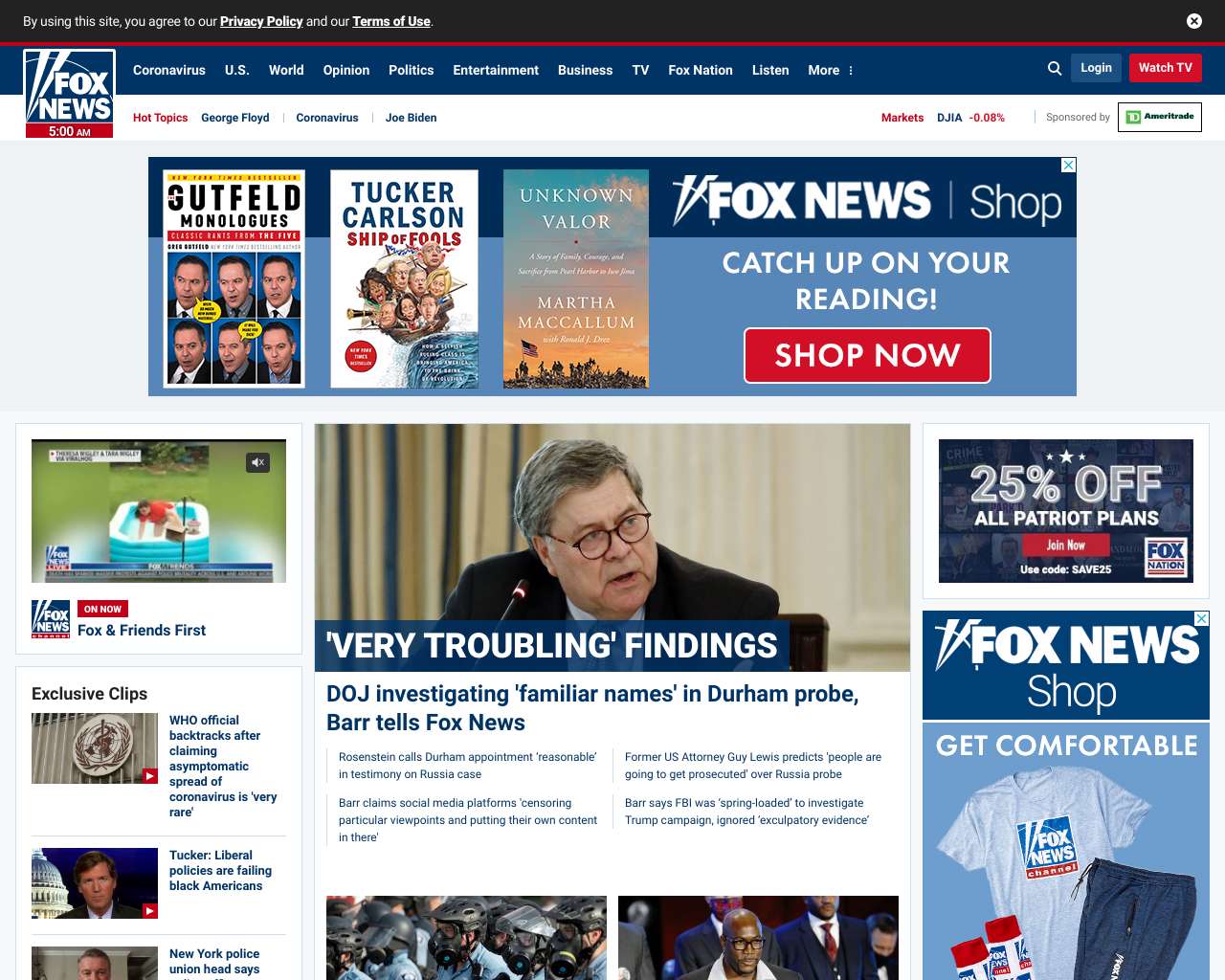The image is a screenshot from a news website showing various sections, advertisements, and articles. Central to the image is a magazine cover titled "Gut-Filled Monologues," featuring six faces. To the right of this, two book titles are prominently displayed: "Ship of Fools" by Tucker Carlson and "Unknown Valor" by Martha McCallum, both available for purchase via Fox News Shop. Additional promotions include a 25% discount on all Patriot Plans with a coupon code and various items such as a t-shirt, pants, and a thermos.

News headlines are scattered throughout the page, including:
- An update on the controversy surrounding the WHO's statement about asymptomatic spread of the coronavirus.
- Tucker Carlson's critique of liberal policies affecting Black Americans.
- Comments from the New York Police Union highlighting troubling findings 
- An ongoing DOJ investigation involving familiar names in the Durham probe.
- Senator Burr's statements to Fox News.

The image also shows an individual dressed in riot gear and another figure, a bald man with glasses in a suit, adorned with a white towel around his neck.

Additional website features include options to log in, watch TV, search, and agree to site policies. An 'X' button at the top right corner offers the ability to close the current pop-up or overlay.